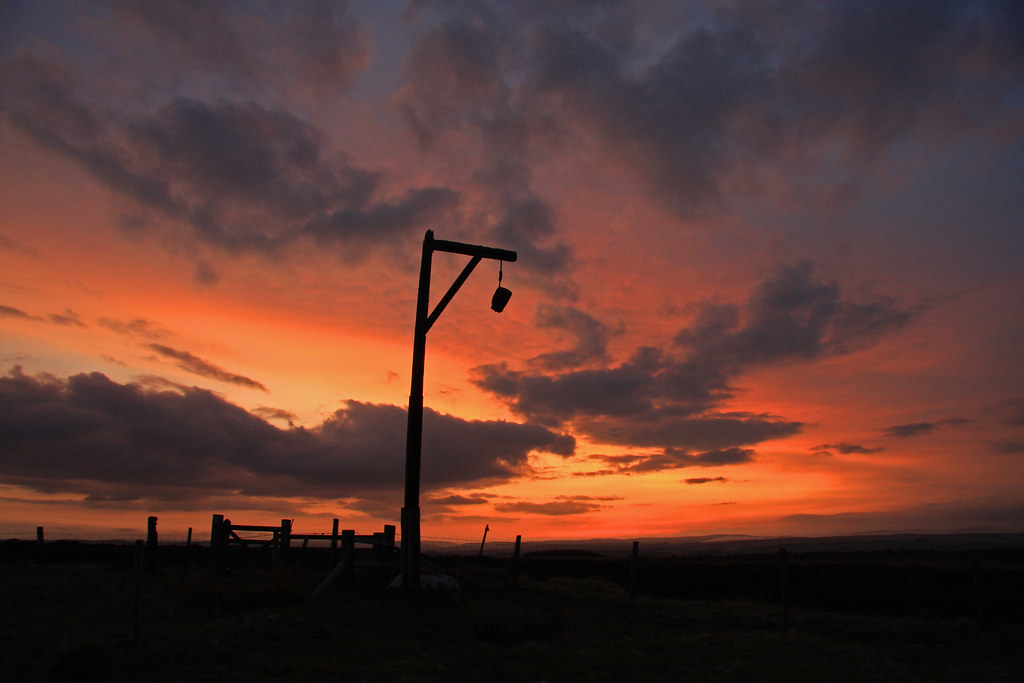The image captures a dramatic sunset with hues of orange, yellow, and red blending into a darker gray-blue sky near the top. Fluffy, purplish-gray clouds scatter across the sky. In the bottom fifth of the image, the foreground is silhouetted, creating a stark contrast against the vibrant sky. A wooden fence, reminiscent of a farm fence, lines the horizon. Central to the foreground, a tall structure resembling an upside-down L creates an imposing silhouette. This structure features a perpendicular board at the top, making a triangular formation with a connecting support beam. From its end, a rope dangles, suggesting a noose or a hanging light, though the silhouetted nature of the object makes it hard to identify exactly what's at the end. This structure evokes the image of a gallows but could also be seen as a light pole. The overall scene is enveloped in the quiet, contemplative atmosphere of the last light of day transitioning to night.